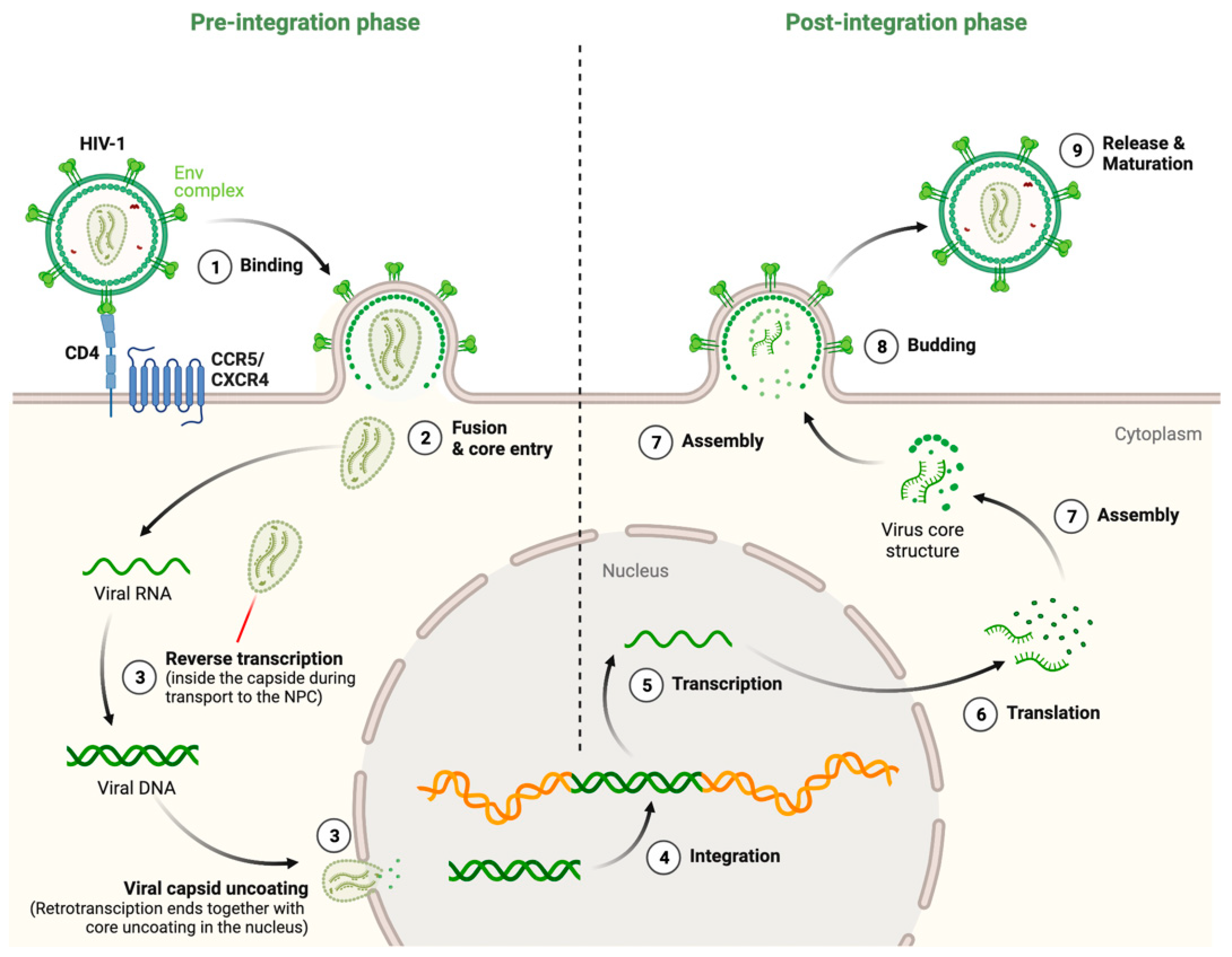This image is a detailed, color-coded diagram illustrating the life cycle of HIV-1 and its interaction with a host cell. The diagram is divided horizontally by a dotted line, separating the pre-integration phase on the left from the post-integration phase on the right. The illustration uses a limited color palette consisting of greens, oranges, blues, and light cream colors to differentiate various elements and processes.

Starting from the top left, the diagram depicts HIV-1 virus particles approaching a host cell. The initial phase, labeled as the pre-integration phase, begins with step 1—binding of HIV to the CD4 protein on the cell membrane. Following this, step 2 illustrates the fusion of the viral envelope with the cell membrane and the entry of the viral core into the cell. Step 3 covers reverse transcription, where the viral RNA is converted into viral DNA by the enzyme reverse transcriptase. 

Arrows guide the viewer through step 4, which is integration, where the viral DNA is inserted into the host's DNA. This marks the transition to the post-integration phase. Steps 5 to 9 sequentially describe the subsequent processes: transcription of viral DNA into RNA (step 5), translation of this RNA into viral proteins (step 6), assembly of new viral particles (step 7), budding of new virions from the host cell membrane (step 8), and finally, release and maturation of the new HIV virions (step 9). Each step is accompanied by illustrative diagrams and numbered for clarity, providing a comprehensive overview of HIV's lifecycle and its replication process within human cells.